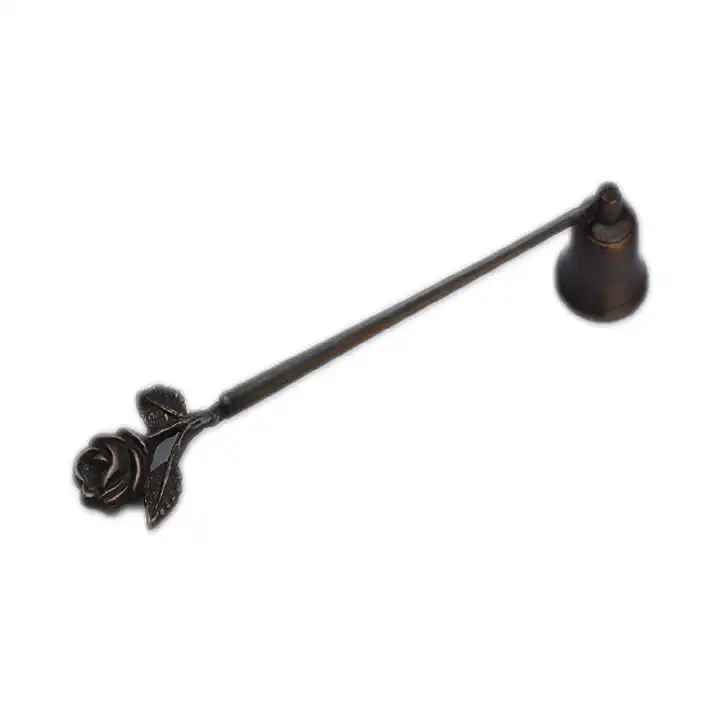The image showcases an antique-style metal candle snuffer with a rich, dark brown to deep rust coloration, resembling bronze or wrought iron. The snuffer features a long, slender handle with a highly detailed rose design, complete with blooming petals and two leaves. The rose, prominently placed on the handle, adds an ornate flair. At the end of the handle, a bell-shaped snuffer is attached via a hinge, allowing it to swivel freely. This bell-like apparatus is designed to extinguish candles by placing it over the flame. The background is plain white, suggesting that the image might be a product photo, possibly for an online store or catalog. The antique quality and intricate design of the rose and leaves lend the piece a ceremonial or collectible aesthetic.